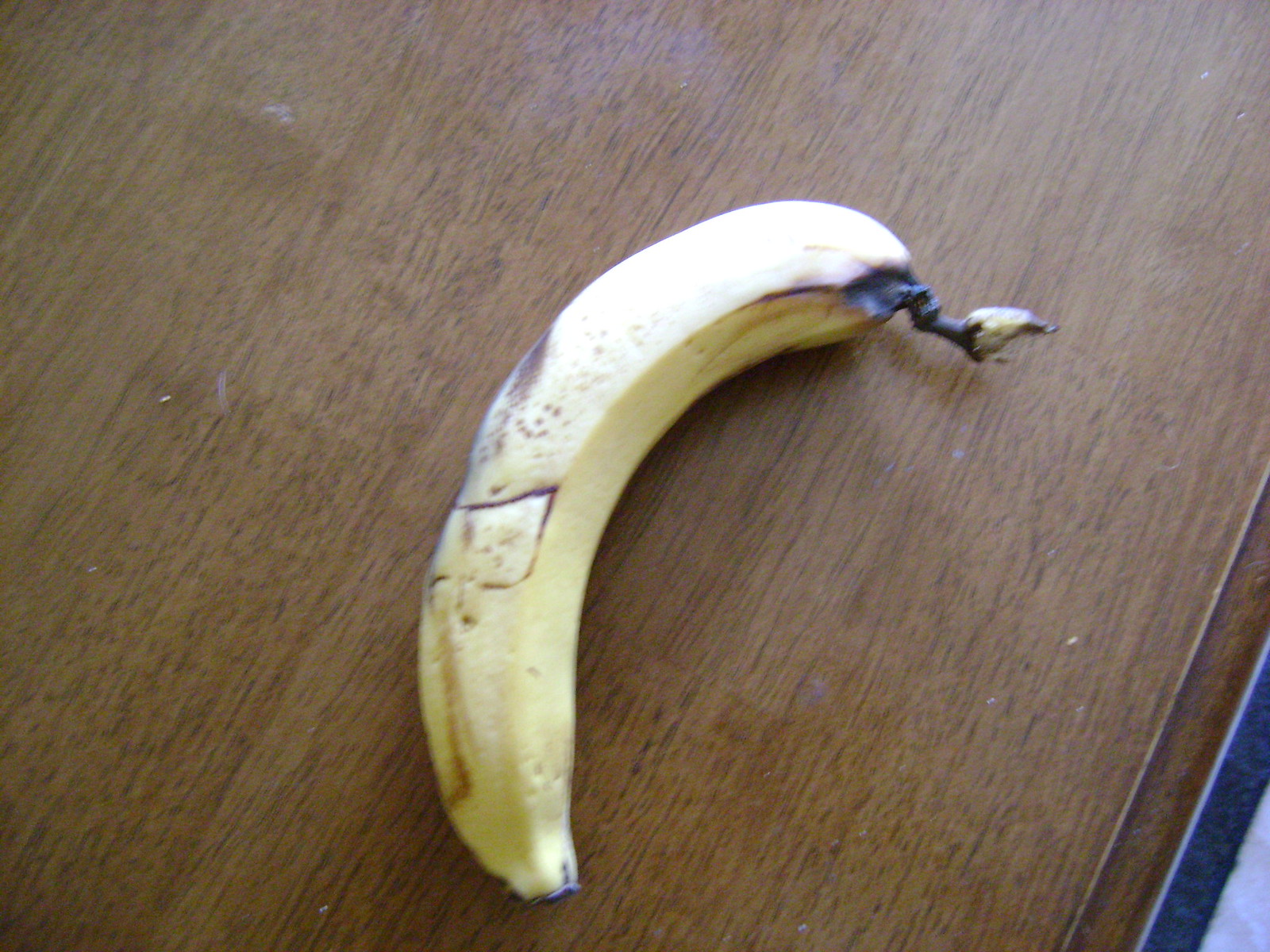A slightly shaky and somewhat blurry image captures a very ripe banana, almost at the point of becoming overripe, resting on a rustic wooden table. The banana, positioned centrally in the frame, displays a gradient of over-ripeness: its top is nearly black, conveying its advanced age, while the lower part appears to be softening and becoming mushy. The lighting in the image suggests daylight, casting a bright natural light over the scene. The worn table surface is not without character, featuring visible dust particles and various stains, enhancing the rustic atmosphere. Towards the lower right corner, a slanted view seemingly exposes a part of the floor, adding to the imagery's casual and unposed nature. No text accompanies the image, allowing the viewer to fully immerse in the visual details presented.